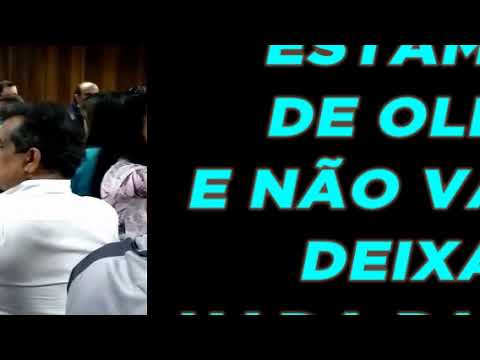The image is a low-quality, out-of-focus screenshot, likely taken from the beginning of a movie or a video seminar. On the left side, there is a narrow, vertically-oriented inset photograph showing a man with dark skin and black hair, wearing a white collared shirt, seated with his back to the camera. To his right, there is a woman in a lavender and white blouse with long black hair. Another man in the back, who is bald with hair on the sides and wearing a black leather jacket, is seated near a wooden wall. The right side of the image has a black background with several lines of bright blue italic sans-serif text in a foreign language. The first row reads "E-S-T-A-M" but appears cut off at the top. The subsequent lines include "D-E-O-L," "E-N-A-O," "V," and "D-E-I-X-A," all partially cut off by the image edge. A dotted line runs horizontally below the text. This chaotic scene, combined with the low light and out-of-focus quality, suggests an informal or candid setting, possibly a gathering or meeting.